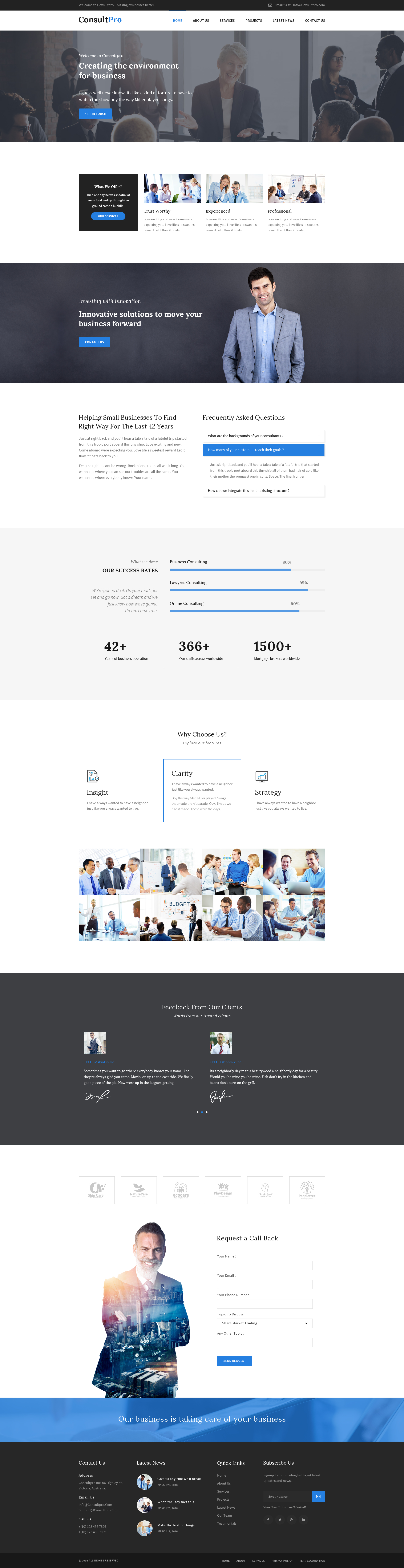The image appears to be a webpage designed for a business that offers motivational or guest speakers for corporate events and collaborations. At the top of the page, there's a faded photograph showing a professional meeting with individuals dressed in business attire, implying a corporate setting.

Below this header image are four clickable tabs or buttons, with the first one currently selected. This section features a prominent, well-dressed man in a suit, likely the keynote speaker or a key figure associated with the service. Accompanying text, though too small to discern, probably highlights the speaker’s achievements and how they can benefit the company.

Further down, there are some statistics indicated by numbers like "42+", "366+", and "1500+", possibly representing audience size, successful events held, or other metrics of success. Blue progress bars are also present, suggesting ratings or levels of accomplishment.

Next, there is a collage of images portraying business activities, predominantly men in suits engaging in discussions and collaborative tasks at meetings. This montage reinforces the professional and corporate nature of the service offered.

Near the bottom section, there are gray boxes, possibly placeholders for additional information or elements such as testimonials or logos. Finally, there's another image, somewhat obscured or creatively altered to appear as if it is viewed through a broken screen or through a filter evoking a sunset, adding a unique visual touch to the webpage’s design.